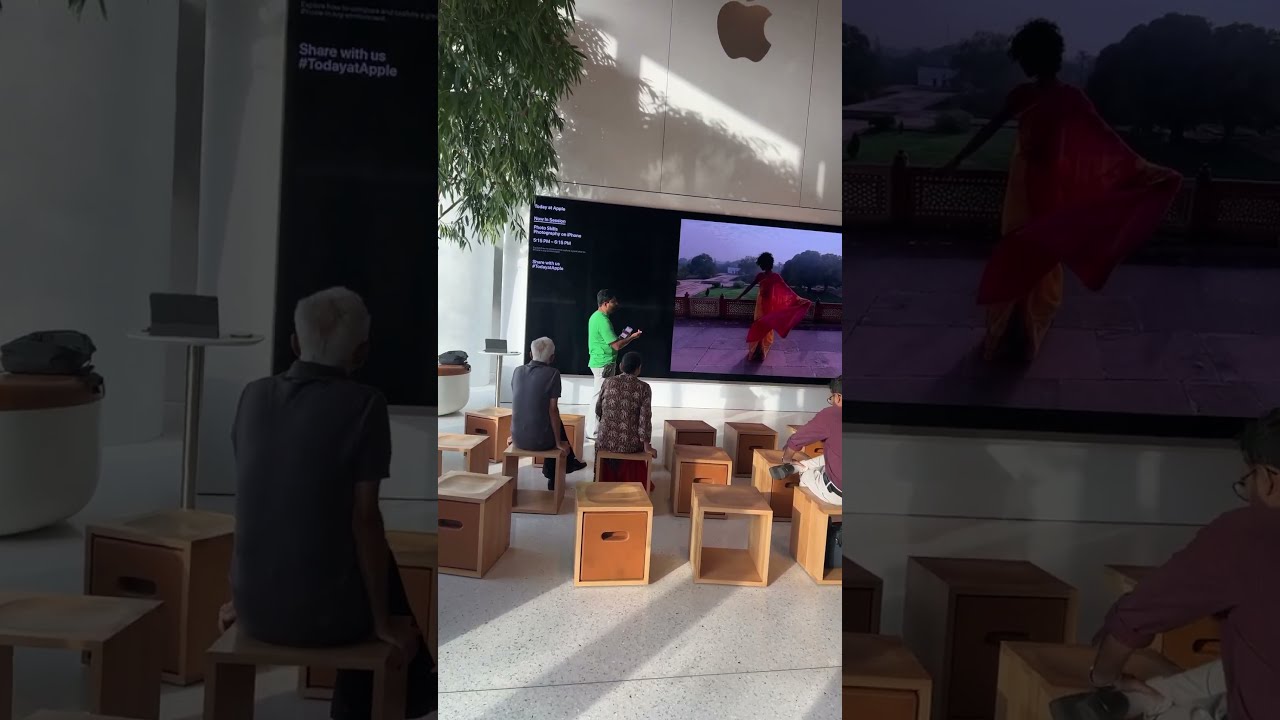The photograph captures a structured meeting or class, characterized by a clear central focus within an intriguing setting. Centered in the middle of the image, participants are seated on unique wooden cube-like chairs with cutouts designed for comfort. Predominantly older, the attendees are focused on a large screen at the front of the room, where a man in a neon green T-shirt and white pants appears to be giving a presentation. The screen displays two main visual elements: a section with text on the left and an image on the right of a woman in a twirling red dress. Adding to the room's professional ambiance is a gold Apple logo situated at the top of the wall, suggesting the setting could be within an Apple office. The floor is covered in a speckled white linoleum, and the room is adorned with a tree, contributing to the unique aesthetic. The photograph, taken through an opening framed by dark glass on either side, also features a faintly grayed-out border inspired by elements of the central image, emphasizing the focus on the described scene.